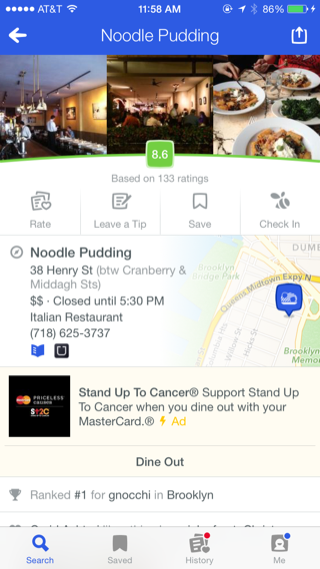A detailed screenshot of a Google search result for the restaurant "Noodle Pudding" features prominently. At the top of the image, a blue bar spans approximately the upper 10% of the screen, displaying navigational and status icons. In the center of the bar, "Noodle Pudding" is written in white text. On the left side of the bar, a white left-pointing arrow suggests a back button, while the right side shows a partially filled green battery icon with a white "86%" next to it, indicating the battery level of the user's phone.

Beneath this blue banner, three photographs related to Noodle Pudding are displayed. One image captures the restaurant's interior, another showcases some of the dishes, and a central photo depicts a large crowd inside the establishment.

Highlighted further down is a green square icon displaying a white "8.6", representing the restaurant's rating. Below this rating, a series of icons with options to rate, leave a tip, save, and check-in are visible.

Continuing downward, detailed information about Noodle Pudding is provided, including the restaurant's name, address, price range, operating hours, classification as an Italian restaurant, and contact phone number.